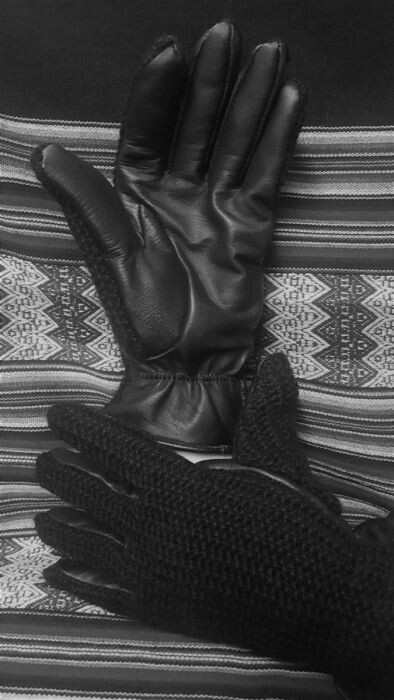In this image, a pair of gloves is prominently displayed against a detailed, multi-textured background. Both gloves are black, with one appearing to be made of smooth, wrinkled leather and the other fabricated from a textured cotton material full of little divots and grooves. The backgrounds showcase varied patterns and colors, featuring jagged shapes and lines in white, maroon, and violet. While the upper portion of the backdrop is entirely black, the main section presents a crumpled or distorted-looking fabric with intricate designs.

The leather glove, positioned right side up, reveals the palm with the thumb pointing to the right. In contrast, the cotton glove is oriented sideways at the bottom of the image, displaying the back of the hand. The overall setting might resemble an indoor scene, possibly on a kitchen table, suggested by the fabric backdrop. The image is in black and white, emphasizing the different textures and details of the gloves against the patterned canvas.